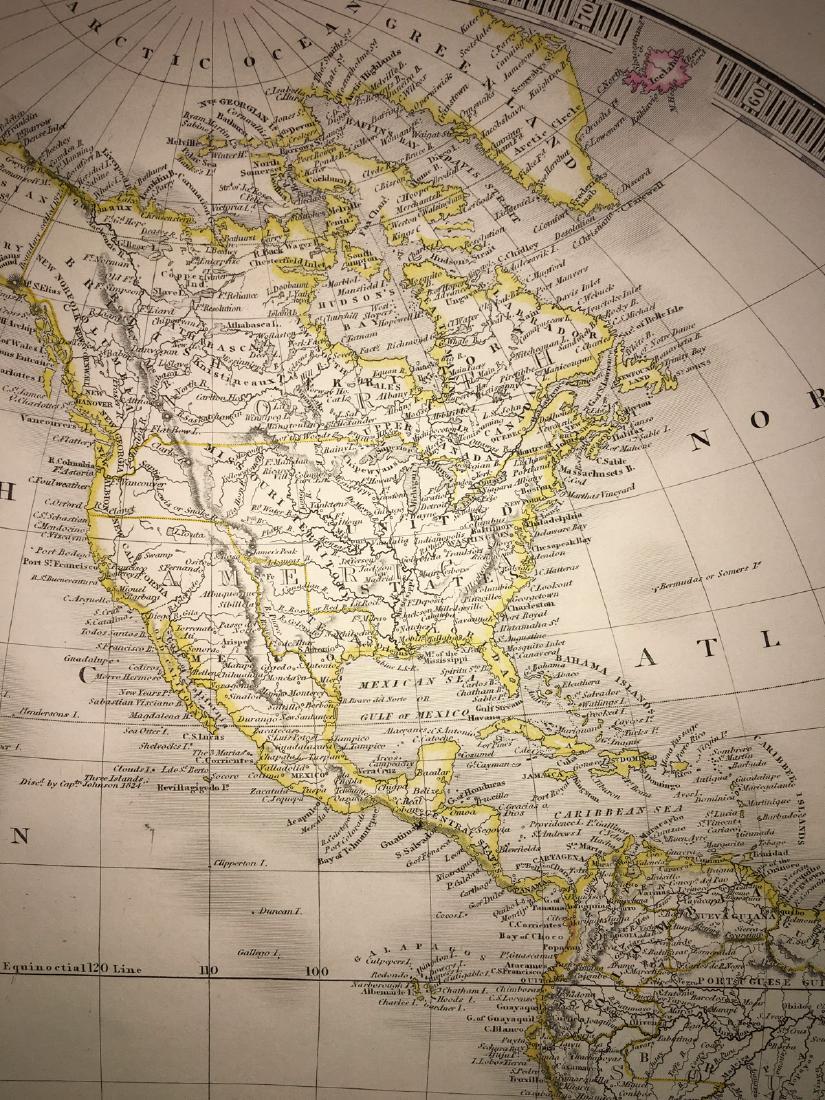This image showcases a detailed, old-fashioned map of North America and parts of South America, displayed on grayish tan or beige paper. The map illustrates the entire North American continent above the northernmost part of South America. Additionally, Greenland and Iceland are present, with borders highlighted in pale yellow and pale pink respectively. Several bodies of water are prominently marked, including the Arctic Ocean and parts of the Atlantic and Pacific Oceans. The Gulf of Mexico is visible between the United States and South America.

The landmasses are outlined in yellow, and all lettering is in black. The map includes intricate and abundant markings, indicating not only regions but also notable areas with old or unusual names, such as "Upper Canada," "Missouri Territory," and "New California." The equator is marked, and despite some modern geographic details, the map contains historical and less-defined territorial labels that extend from Canada down to the equinox line. The presence of the Mexican Sea is noted, along with the smaller islands, including Cuba. Overall, the map is rich in detail and historical references, a testament to the intricate cartographic work of the period.